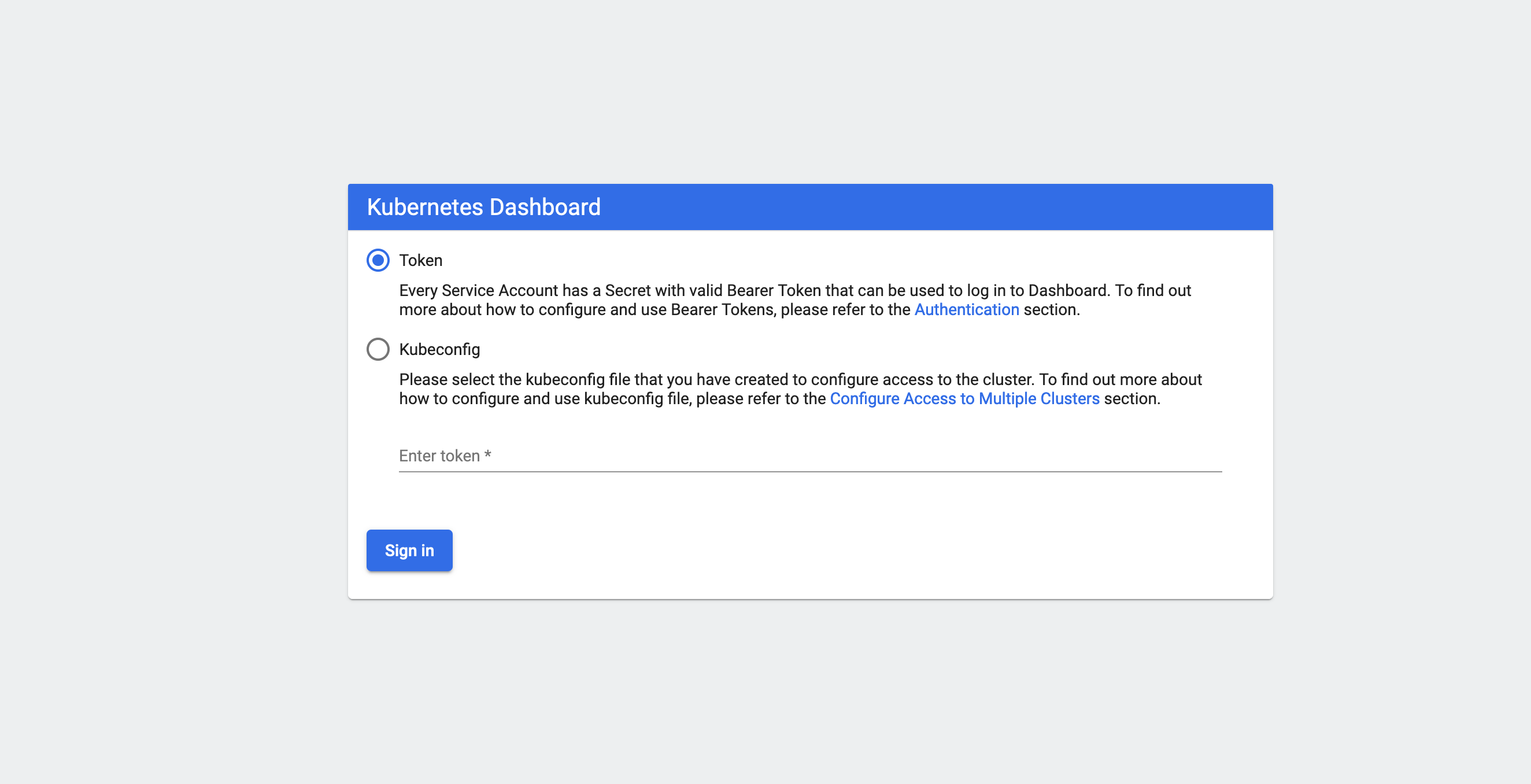The image displays a screenshot of a computer application, specifically the Kubernetes Dashboard interface. The background of the image is a plain, flat gray. In the center, there is a white rectangular dialog box with a blue header. The header features the text "Kubernetes Dashboard" in white font.

Within the dialog box, on the left side, there are two main sections for authentication options. 

1. **Token Authentication**:
   - This section is marked with a blue circle indicating that it is the selected option.
   - The text reads: "Every service account has a secret with a valid bearer token that can be used to log in to the dashboard. To find out more about how to configure and use bearer tokens, please refer to the authentication section."

2. **Kubeconfig Authentication**:
   - This is the secondary option and is noted by an unselected circle.
   - The accompanying instruction is: "Please select the kubeconfig file."

Below these sections, there is a line separator. Above the line, it says "Enter token" followed by an asterisk, indicating a required field.

To the right, there is a "Sign In" button, which remains within the white rectangular box.